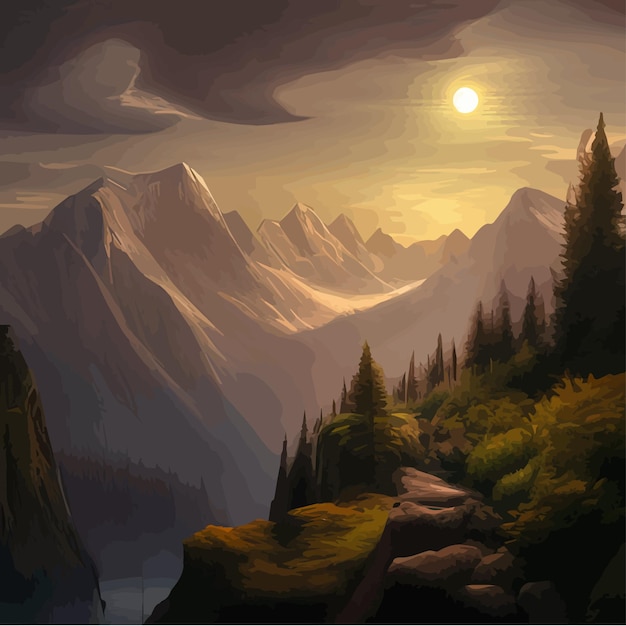This digital artwork captures the essence of nature and wildlife through a detailed, mountainous landscape. The foreground, located on the bottom right, features a lush hillside covered in pine trees, evergreens, bushes, moss, grass, and various boulders. The landscape is rich in vibrant and contrasting colors: deep greens, browns, and grays. As your eye moves towards the distance, the painting reveals a range of mountains, whose peaks appear snow-capped and hazy, rendered predominantly in grey tones. Above, a bright sun, glowing with white and yellow radiance, illuminates the otherwise grey sky, casting light on the cloud-covered expanse. The overall artwork gives a sense of serenity and raw natural beauty, blending elements of concept art and digital filtering to separate similar colors into distinct bands and shapes, making the scene both intricate and picturesque.